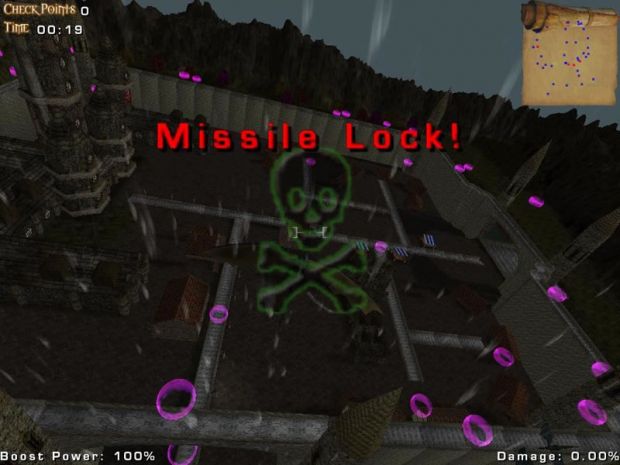This screenshot from a video game displays a dark, futuristic scene dominated by shades of black and gray. Central to the image is a green skull and crossbones with the warning "MISSILE LOCK!" prominently displayed in red text above it. The top left corner of the screen features the word "Checkpoints" in yellow, with a timer beneath it indicating "00:19" in white font. On the top right, there is a scroll-like map with purple and red dots, likely indicating the player's position and objectives. Scattered throughout the screen are several purple ring-shaped circles. The bottom left corner shows "Boost Power 100%" in white, while the bottom right corner details "Damage: 0.00%" in tiny font. The setting includes a maze-like, black area fenced in the center, some jagged rock formations or possibly city structures in the background, and a few buildings within the maze. Tall, cylindrical structures that resemble missiles can be seen in the upper left corner.